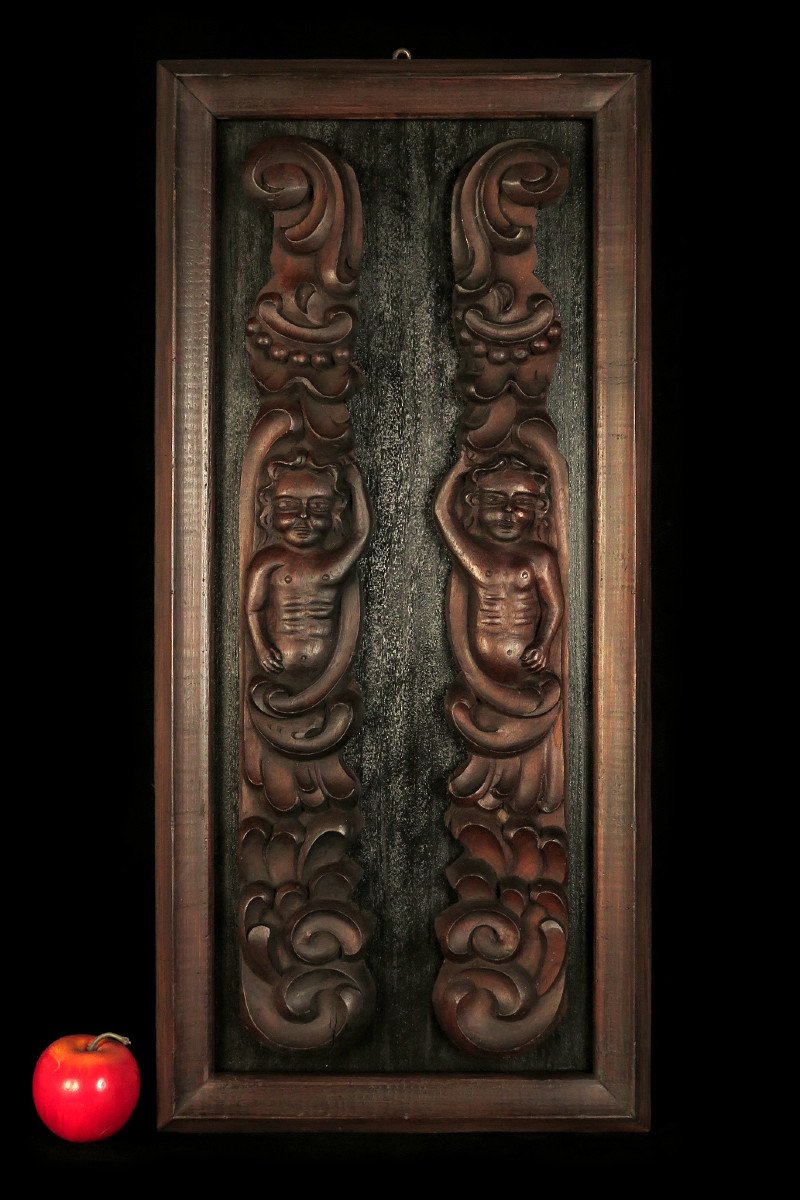The framed artwork features intricate wooden carvings set in a dark brown, antique wood frame with a metallic circular hoop for hanging. The piece is vertically oriented, taller than it is wide, with a black, textured background. Within the frame, there are two almost identical human figures carved from medium brown wood, positioned like columns with ornate, wave-like designs at the top and bottom. These figures, reminiscent of totem poles, are depicted with one arm raised and the other down by their side. A striking detail is a shiny red apple with a bit of a stem located in the left-hand bottom corner, set against the black background as if floating without a visible surface to rest on. The overall piece has a curious and mysterious aesthetic, blending traditional and whimsical elements.